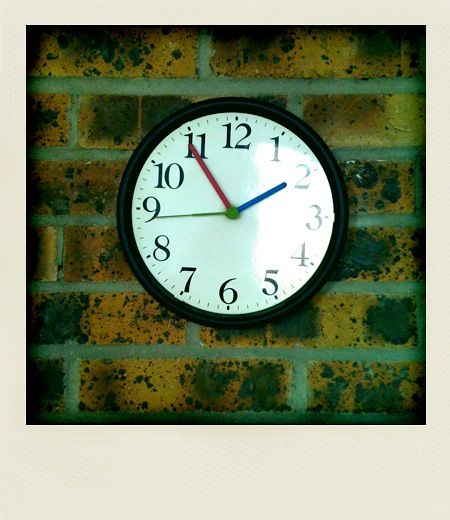A framed clock hangs against a backdrop of a weathered brick wall, characterized by brick patterns interspersed with gray concrete lines, and black splotches adding to the aged appearance. The clock itself sports a sleek black body and a reflective clock face, subtly catching light on the right side. Notably, the clock features distinctive colored hands: a red minute hand pointing to 11, a blue hour hand at 2, and a green seconds hand at 9. Surrounding the clock face are dash marks, and numerals from 1 to 12 arranged in a traditional clockwise direction.